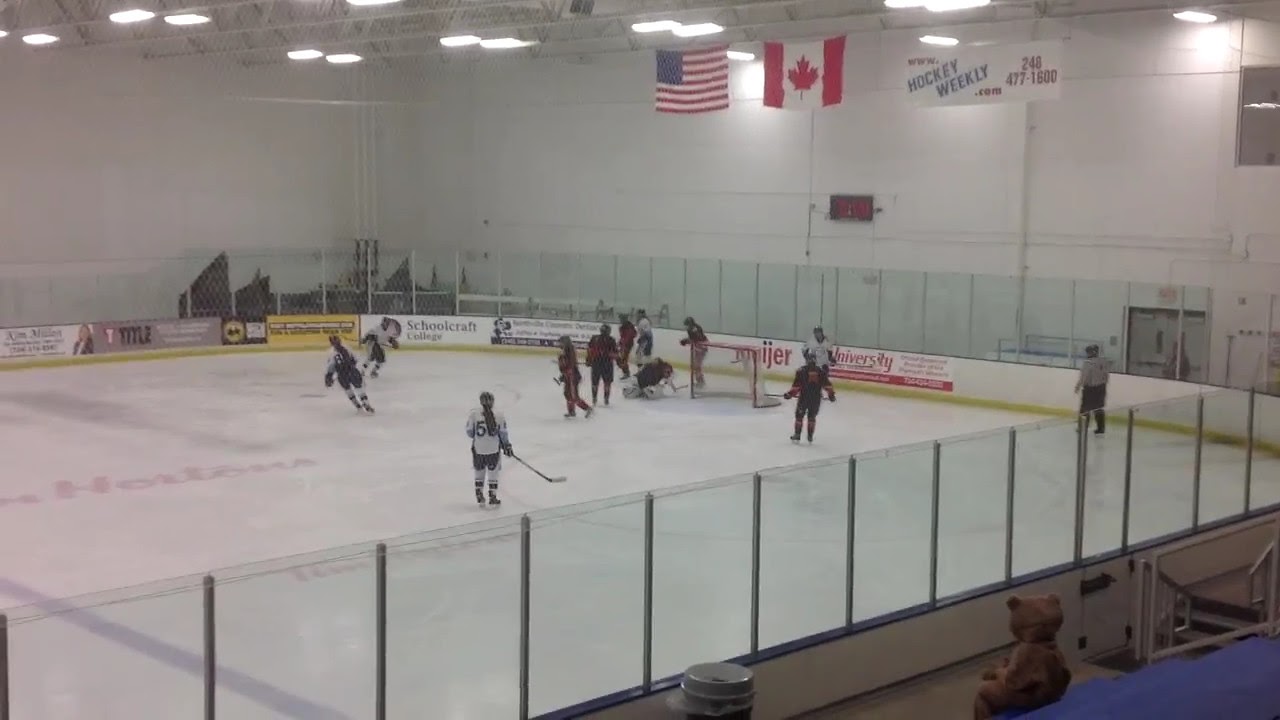The photograph captures an intense girls' hockey game inside a nondescript rink, with players skating energetically across the ice. The two opposing teams are distinguishable by their uniforms—one team is clad in white while the other wears black and red. The image is taken from higher up in the bleachers, providing a view of most of the rink and one of the goals. Hanging above the rink are both American and Canadian flags, alongside a banner that reads "Hockey Weekly" with the website www.hockeyweekly.com and the phone number 248-477-1600. The arena's walls are unadorned white, accented only by several flags and banners, including advertisements for Meyer and Schoolcraft College. A character in a brown bear costume, likely a team mascot, and another individual wearing a gray cap can be seen among the spectators in the bleachers. The vibe is lively and competitive, emphasizing the spirit of the sport.